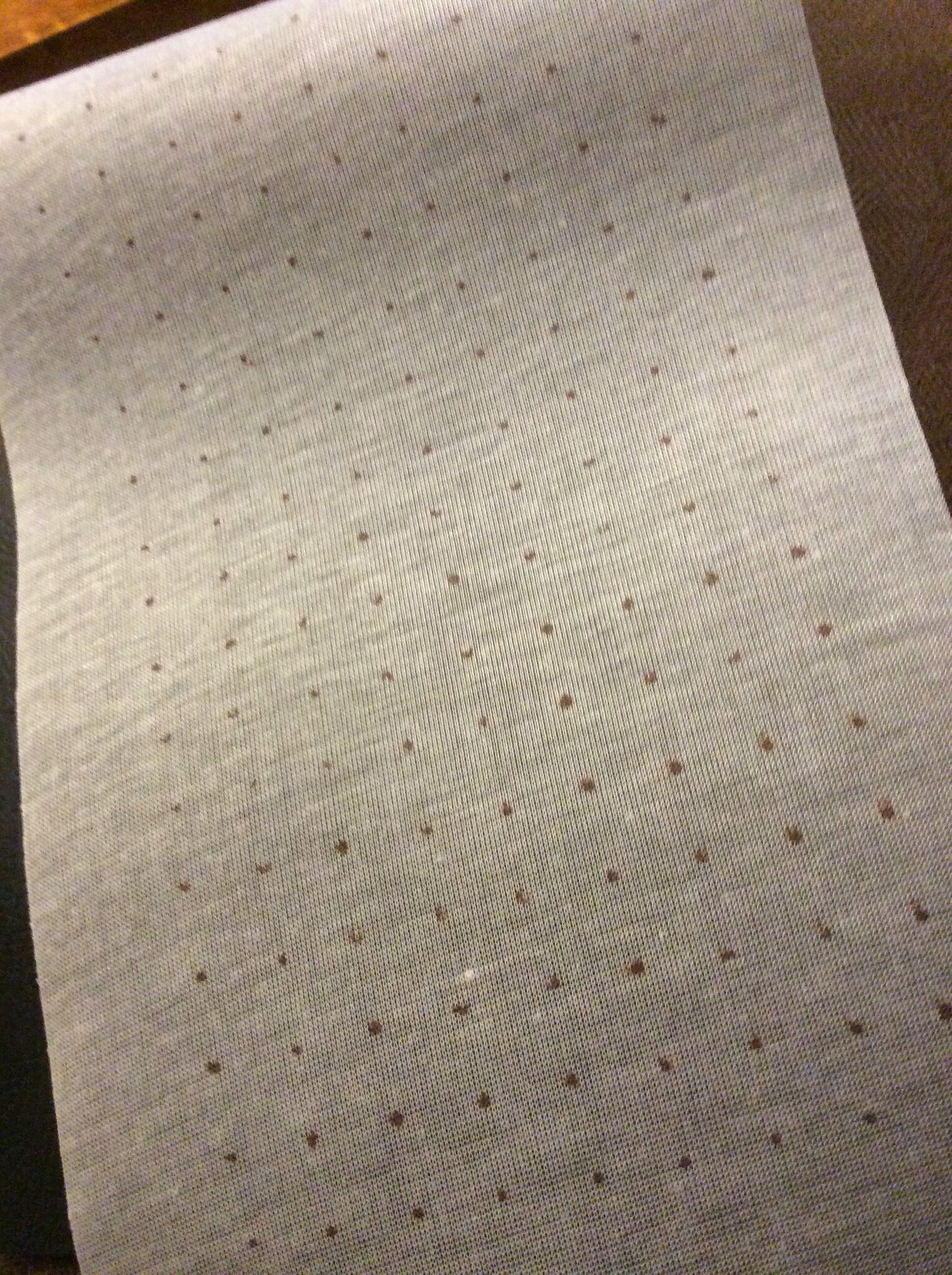This is a portrait-oriented photograph of a piece of light beige linen or tightly woven fabric. The cloth is beige to off-white in color and features small brown dots arranged in parallel rows and columns, covering the entire visible surface. The dots are evenly spaced, with nine dots across and at least sixteen dots down the length of the fabric. Borders can be observed on either side of the cloth, creating a space between the edge and the first row of dots. The fabric appears to have a slight wave, suggesting it had been rolled up and then unrolled, with noticeable undulations near the middle and a more pronounced wave at the top. The cloth seems to be placed on a darker brown surface, perhaps furniture or a couch, which appears darker at the bottom left and lighter towards the upper right. The photo is closely cropped, preventing the bottom edge of the fabric from being visible.